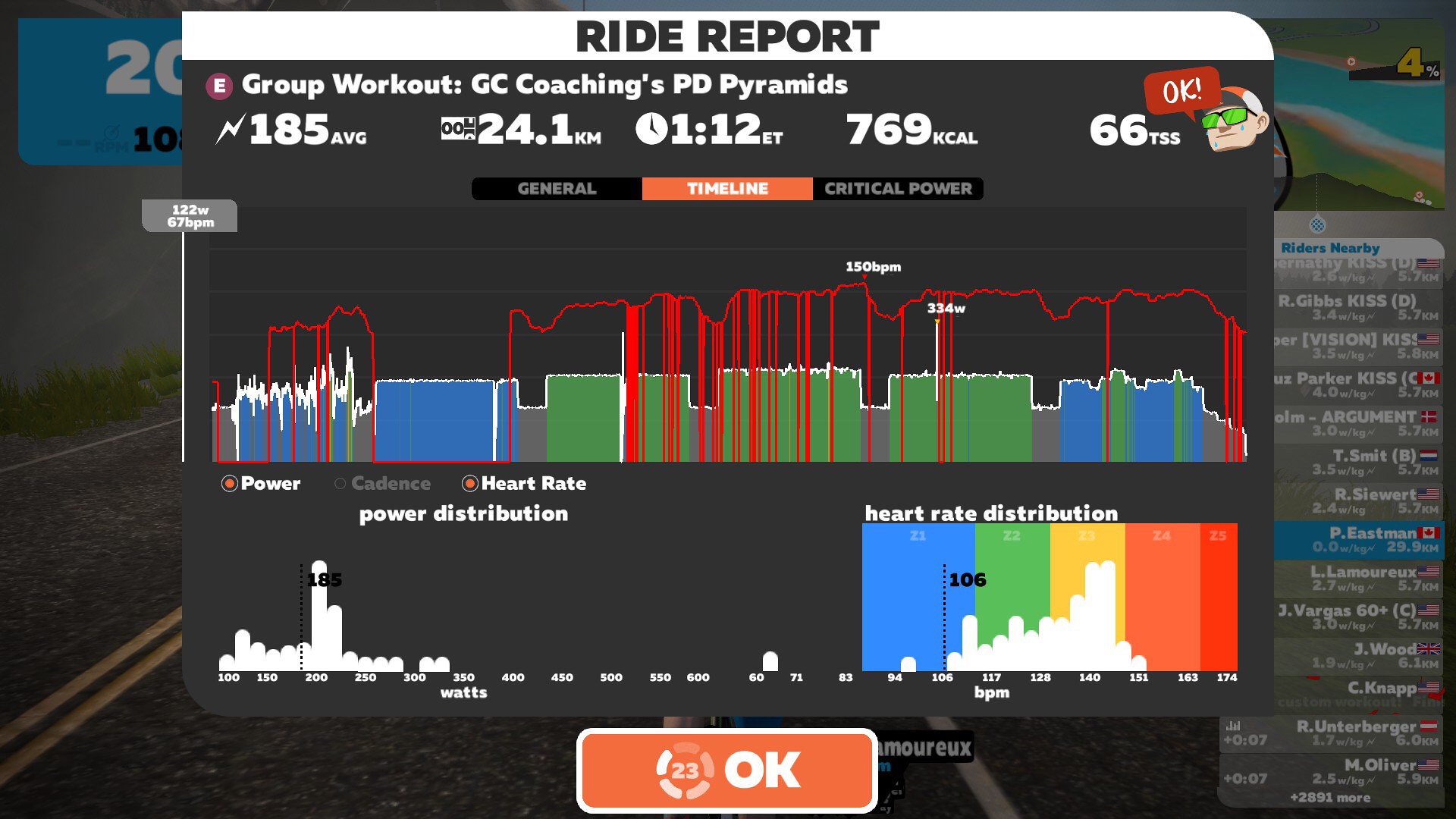The image is a detailed "Ride Report" from a fitness tracking application, set against a vague background of a street with yellow lines. At the top, it prominently features a maroon circle with a white letter "E" beside the text "Group Workout: GC Coaching, PD Pyramids." Adjacent to this, there's a white lightning bolt symbol followed by "185 Average," a white circle with black zeroes and "24.1 KM," a clock icon with "112 ET," the numbers "769 KCAL," and "66 TSS" beside a cartoon character wearing green sunglasses, a white and orange cap, and displaying blue sweat drops.

Below this header are three centered rectangles, labeled "GENERAL," "TIMELINE" (in orange), and "CRITICAL POWER." Beneath these headings, grid charts display metrics like "Power," "Cadence," and "Heart Rate," color-coded from blue to green to yellow to orange to red, indicating varying levels of heart rate distribution. Within the grid, you see detailed statistics, such as "122W" and "67 BPM." The bottom third features two additional graphs spanning the width of the report: "Power Distribution" on the left and "Heart Rate Distribution" on the right. The bottom-left corner graph measures power in watts, while the bottom-right graph categorizes heart rate data using the same color codes mentioned earlier. At the very bottom is an orange rectangle with "OK" in white, and a circle containing the number 23.